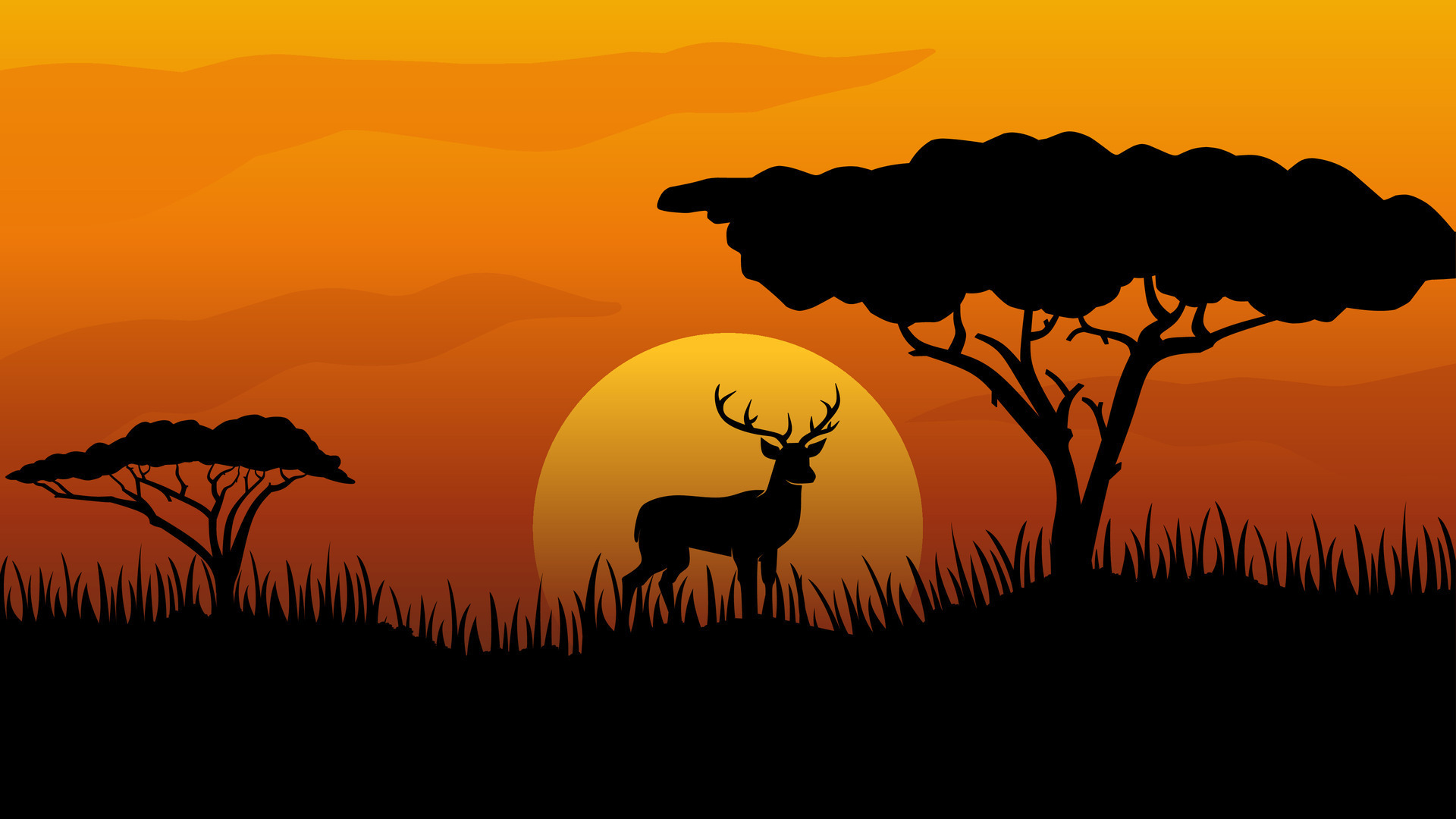In this simplified, yet evocative color drawing, we see an African savannah setting during what appears to be either sunrise or sunset. Dominating the bottom fourth of the image is a completely black, silhouette-style terrain featuring grass and two distinct flat-topped trees with stark black trunks. The grass, portrayed in a mix of tall and short blades, creates a ticker-tape like horizon. A stag with a prominent six-point antler rack stands in the center of the scene, gazing to the right. Behind the stag, an orange disc signifies the Sun, transitioning from a light yellow at its apex to darker hues toward its base. The sky above is a gradient of light to dark orange, with purple undertones, and is scattered with a few darker areas symbolizing clouds. The scene's overall design is a striking contrast of vivid background colors against the silhouette foreground, lending a serene yet dramatic atmosphere to the artwork.